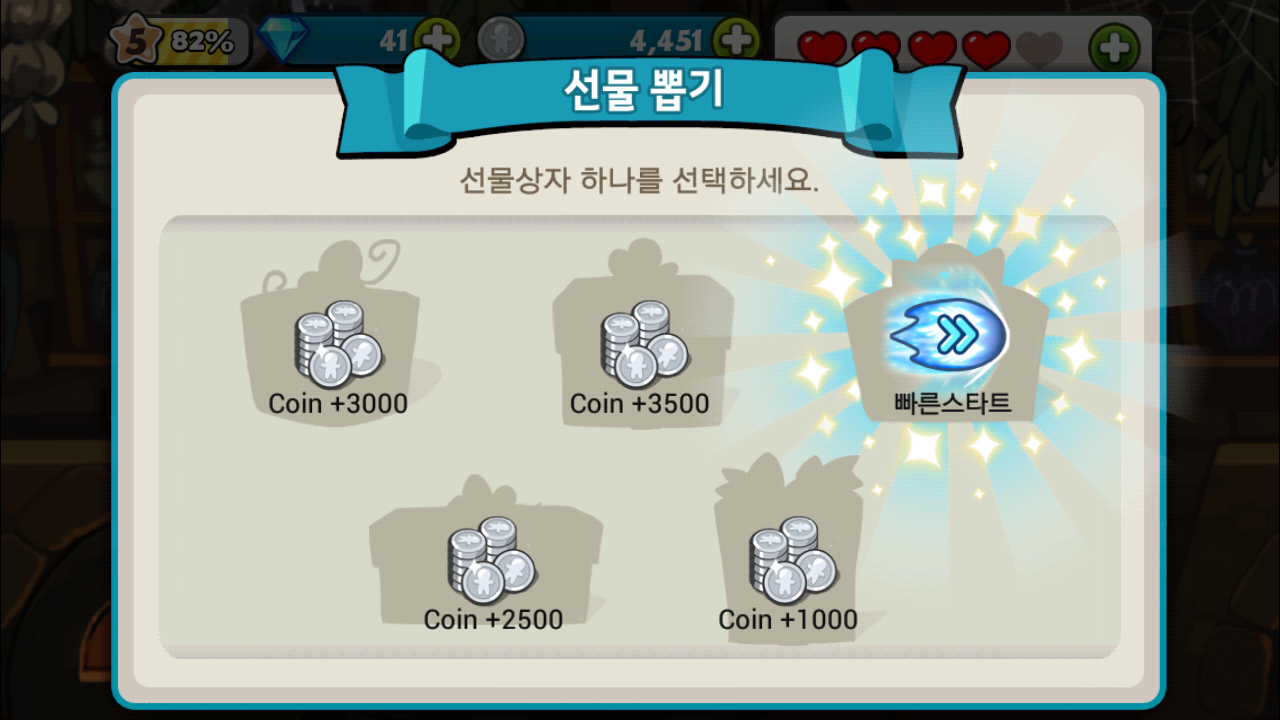The image depicts a screenshot from a mobile game screen, predominantly featuring a cash-out prize menu with different coin amounts. The top of the screen displays a blue banner with white Chinese characters, followed by another set of brown Chinese characters underneath. Positioned nearby are a star icon with the number "5" and an "82%" label, a little gem symbol with a "41" and a green plus sign, and a figure "4451" followed by four red hearts and a plus sign.

Just below these elements, the main part of the screen shows five different cash-out options, each accompanied by a coin icon. The prizes include:
- Coin +3,000
- Coin +3,500
- Coin +2,500 (bottom left)
- Coin +1,000 (bottom right)

Additionally, there is another icon with a power-up symbol and Chinese characters. One of the options, highlighted with stars and blue streaks, seems to be activated or won, implying its significance in the game. The overall visual design includes gray, white, and teal colors, consistent with the aesthetic of a typical mobile game interface.